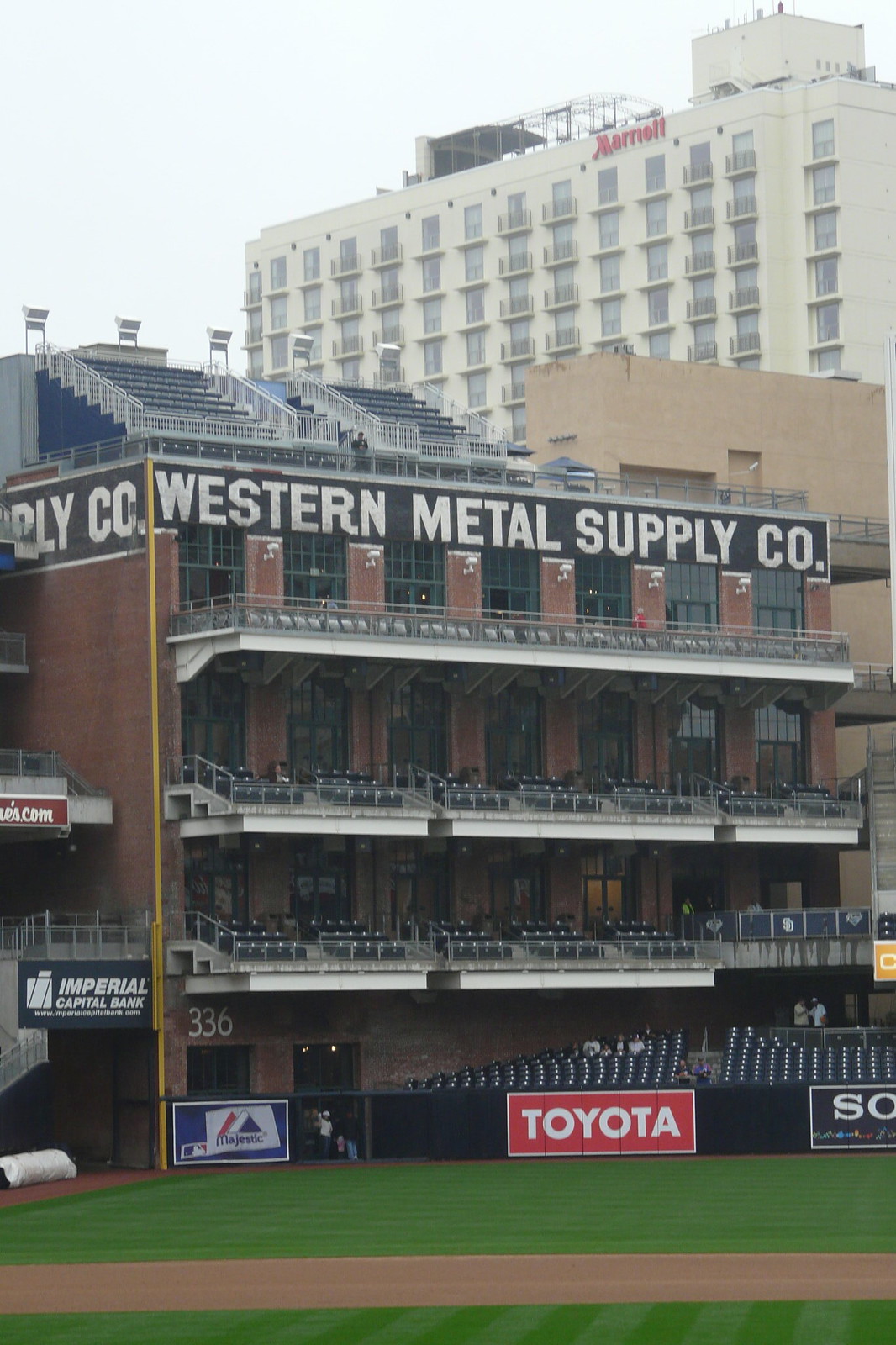The photograph captures a vibrant baseball field set against a cloudy sky, with a range of advertisements prominently displayed. In the foreground, the green expanse of the field is bordered by a dirt track. Beyond the field is the Western Metal Supply Co. building, a striking four-story red-brick edifice featuring black balcony seating on the top three floors and additional bleacher seating below, all secured behind a tall chain-link fence. The building’s façade bears a notable black box sign with white font reading "Western Metal Supply Company."

Along the field's border, various advertisements are visible: "Imperial Capital Bank," "Toyota," and "Majestic." Behind the Western Metal Supply Co. building looms the Marriott Hotel, a towering skyscraper with numerous glass windows and beige coloring, which provides a striking background to the scene. In front of the field, spectators can be seen sitting in the seats and standing around, contributing to the lively atmosphere of the baseball stadium. The palette of colors in the image includes greens, browns, beiges, blues, blacks, grays, and whites, enhancing the complexity and detail of the overall scene.